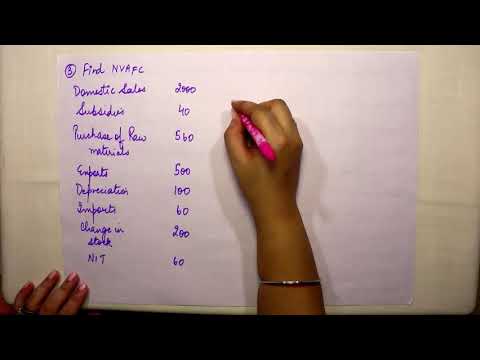In this top-down image, which appears to be a screenshot from an instructional video, we see a detailed view of a woman's hands engaged in note-taking on a large white piece of paper. The woman writes with a pink pen that produces purple ink. Her right hand, adorned with a silver bracelet, firmly holds the pink pen between her thumb and index finger, while her left hand steadies the paper. The paper contains various business-related content written in cursive, including terms and statistics such as "Find NVA FC," "depreciation," "purchase of raw materials," and several monetary values like "domestic sales, $2,990," "subsidies, $40," and "purchase of raw materials, $560." The scene suggests that the notes pertain to instructional material, likely for an accounting or business class, with the paper placed on a desk or similar surface.